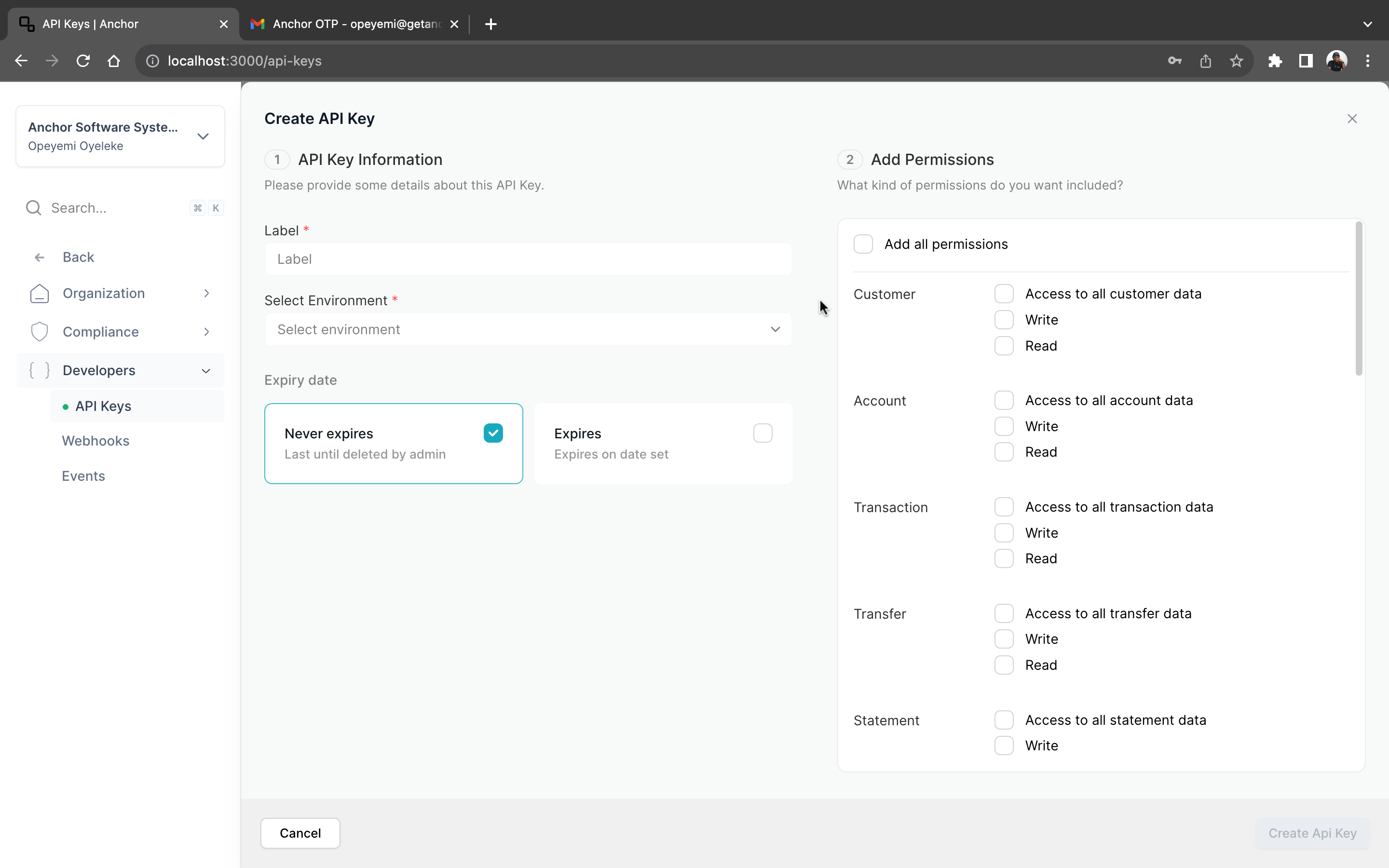Screenshot of a browser window with two visible tabs. The first tab, labeled "API keys | anchor," displays a management interface for API keys. The second tab, noted as "anchor OTP," appears to be a Gmail inbox for the Anchor service. The primary focus is on the "anchor software system" interface.

On the left sidebar, options such as "Organization," "Compliance," and "Developers" are visible, with subcategories under "Developers" including "API Keys," "Webhooks," and "Events." The main screen is dedicated to creating a new API key. Users are prompted to enter details such as the label, environment, and expiry date for the API key, with options for "Never Expires" or "Expires."

To the right of the API key creation section, there is an "Add Permissions" segment, where users can assign permissions either universally ("Add All Permissions") or individually. Specific permissions categories include "Customer," "Account," "Transaction," "Transfer," and "Statement," with each category allowing granular control over data access (read, write, or all).

The interface features a clean, minimalist design with a color scheme of white, light gray, and dark gray. The only hint of color comes from a tiny, partially obscured Gmail logo on the second tab.